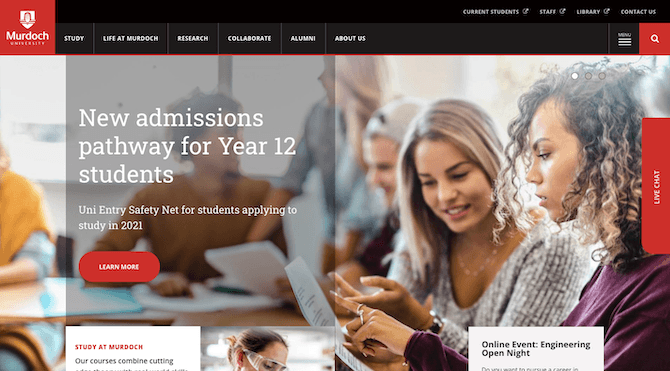This image captures a detailed screenshot of a webpage, presumably the homepage of Murdoch University’s website. The web address, browser, and operating system are not visible. 

In the top left corner, there is a prominent red square featuring white text and a white shield emblazoned with an emblem that is too small to discern clearly. The name "Murdoch University" is written beneath the shield.

A black menu bar extends across the top of the page with white text options including:
- Study
- Life at Murdoch
- Research
- Collaborate
- Alumni
- About Us

In the top right, several clickable pop-out windows provide access to various sections of the website, such as "Current Students," "Staff," "Library," and "Contact Us." A hamburger icon, represented by three horizontal bars, and a red search box are also located in this area for easy navigation.

Below the menu bar, a central image depicts several individuals seated at a table. All are dressed in long sleeves, suggesting a cold environment. The group appears to consist mostly of women with one man, and they seem to be in their early 20s, focusing intently on papers before them.

Overlaying this image in white text is the message: "New Admissions Pathway for Year 12 Students, Uni Entry Safety Net for Students Applying to Study in 2021." Additionally, a red pill-shaped button with white text invites users to "Learn More."

Lower on the page, a woman wearing safety goggles is visible, indicative of a hands-on or scientific activity. Adjacent red text promotes studying at Murdoch with partially visible lines including "Study at Murdoch," "Our Courses," and "Combined Cutting," though some text is cut off. To the right of her image, another partially visible heading reads: "Open Event, Engineering, Open Night. Do you want to pursue a career in," though this text is also truncated.

Overall, this screenshot provides a comprehensive overview of Murdoch University’s homepage, highlighting key navigation elements, an informative central banner, and a glimpse into the university’s promotional events and study options.